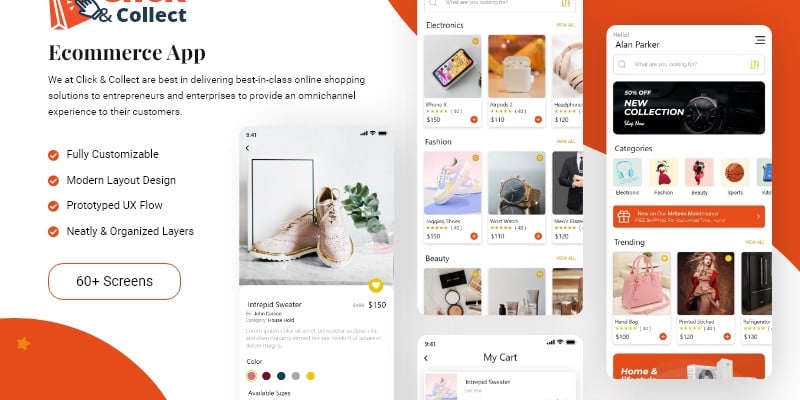This image represents the layout of an e-commerce application website named "Click and Connect". The website's header highlights their expertise: "We at Click and Connect are best in delivering best-in-class online shopping solutions to entrepreneurs and enterprises to provide an omnichannel experience to their customers." Beneath this statement, a list is displayed with orange check marks that signify the key features of the platform: fully customizable, modern layout design, prototyped UX flow, neatly organized layers, and over sixty screens.

To the right of this text, a screen showcases a sneaker with its price prominently displayed. Adjacent to this, another screen features a variety of product images from different categories such as electronics, fashion, and beauty. At the bottom, there's a "My Cart" section with thumbnail images beside listed items, each showing the respective prices.

On the far right side of the layout, the name "Alan Parker" is displayed at the top, followed by sections labeled "New Collection," "Categories," and "Trending," indicating additional items available for sale. The website employs a color palette consisting of orange, white, gray, pink, blue, black, and yellow to create a visually engaging and functional design.